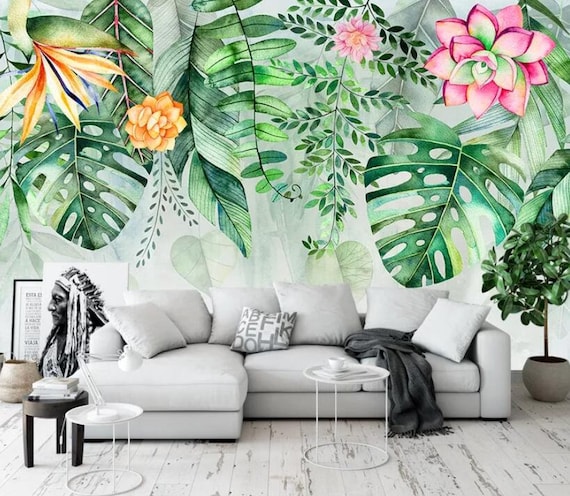The image depicts a stylish and cozy indoor space centered around a large, L-shaped white sectional couch adorned with many white cushions. Among these cushions, one pillow stands out with gray letters scattered across its white fabric. The couch is flanked on the left by a dark gray blanket and to the right by a potted green tree. The couch rests on white-paneled flooring, which has small scrape marks, giving it a slightly rustic charm.

Above the couch, the wall is covered with a botanical-themed wallpaper featuring varying shades of green leaves, interspersed with pink, orange, and yellow flowers of different sizes and shapes. Notably, an orange flower in the top left corner bears a striking resemblance to the head of a peacock or parrot.

In front of the couch, there are two white circular coffee tables, and on the right side of the couch stands a similar white table with a white lamp on it. Additionally, a black table to the right holds a few objects. The decor includes a notable black and white artwork of a Native American man in a headdress, accompanied by another piece featuring an array of words. The overall aesthetic is accentuated by clean lines, soft colors, and natural elements, creating a harmonious and inviting atmosphere.